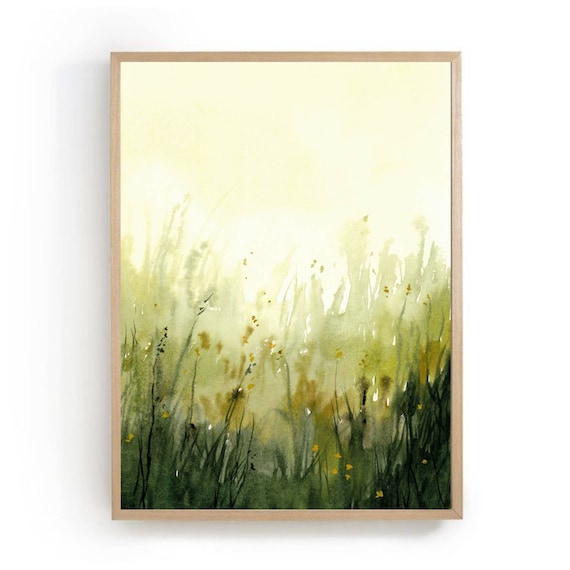This is a depiction of a framed watercolor painting set against a white wall background. The frame, likely made of wood, has a beige tone, casting a slight shadow beneath it. The painting is primarily composed of bright yellows and muted greens, creating a vibrant yet soft and abstract meadow scene. The lower portion is filled with an array of small plant branches, leaves, and perhaps blossoms, evoking an early morning atmosphere with a touch of misty dew. The upper section fades into a wash of yellow and white, reminiscent of a morning sky. Though the flowers and plants are not distinctly clear, the abstract arrangement suggests a natural, serene landscape.